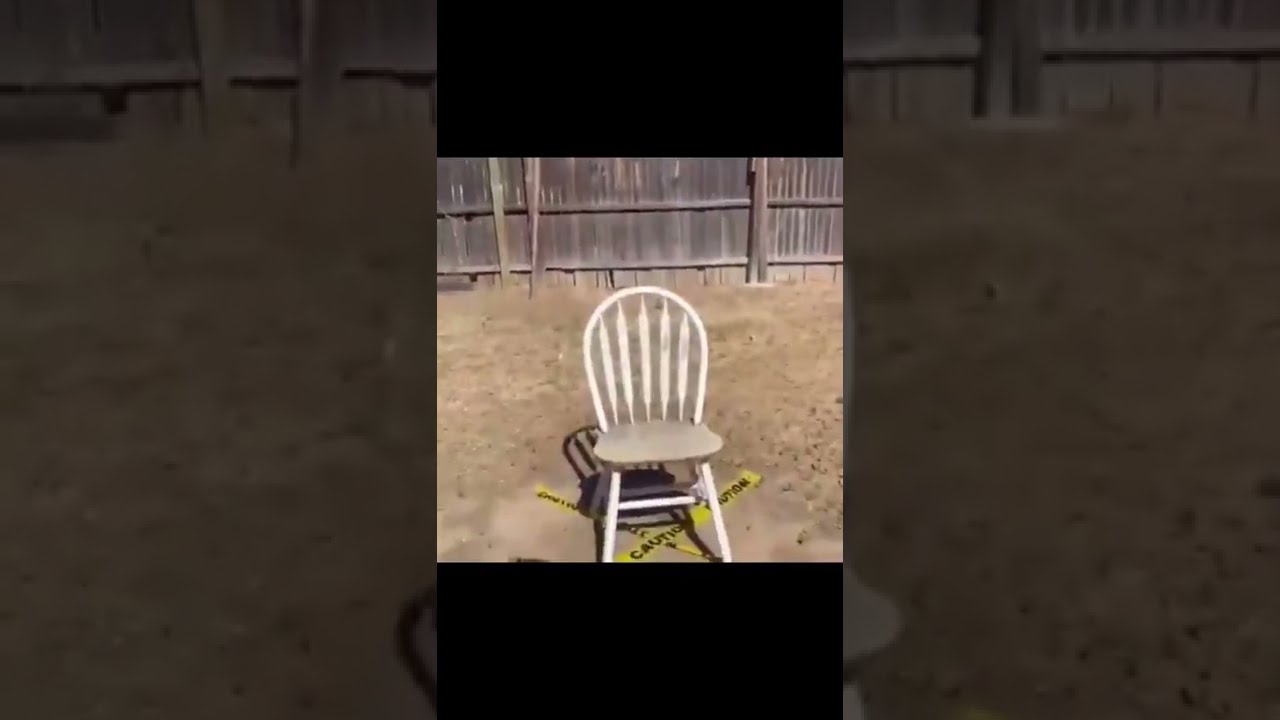This detailed photograph features a weathered white wooden chair positioned in a dirt yard, bordered by an old and unpainted wooden fence. The image is segmented into thirds, with the left and right thirds highlighting zoomed-in sections of the central scene, making the central portion the primary focus. The central section is letterboxed at the top and bottom, encompassing about 25% each, to emphasize the main subject — the chair. The chair's paint is chipped, revealing a grayish tint on its flat seat. Despite its deteriorated state, it stands with four legs and has a backrest with vertical spokes arching at the top. Beneath the chair, pieces of yellow caution tape intersect, forming a V. The backdrop extends into a bare dirt yard, hinting at a bygone lawn, and culminates in a weather-beaten fence. The zoomed-in left and right thirds, faded to half opacity, reiterate the continuous expanse of dirt and the rustic fence, framing the neglected chair at the core of this desolate outdoor setting.